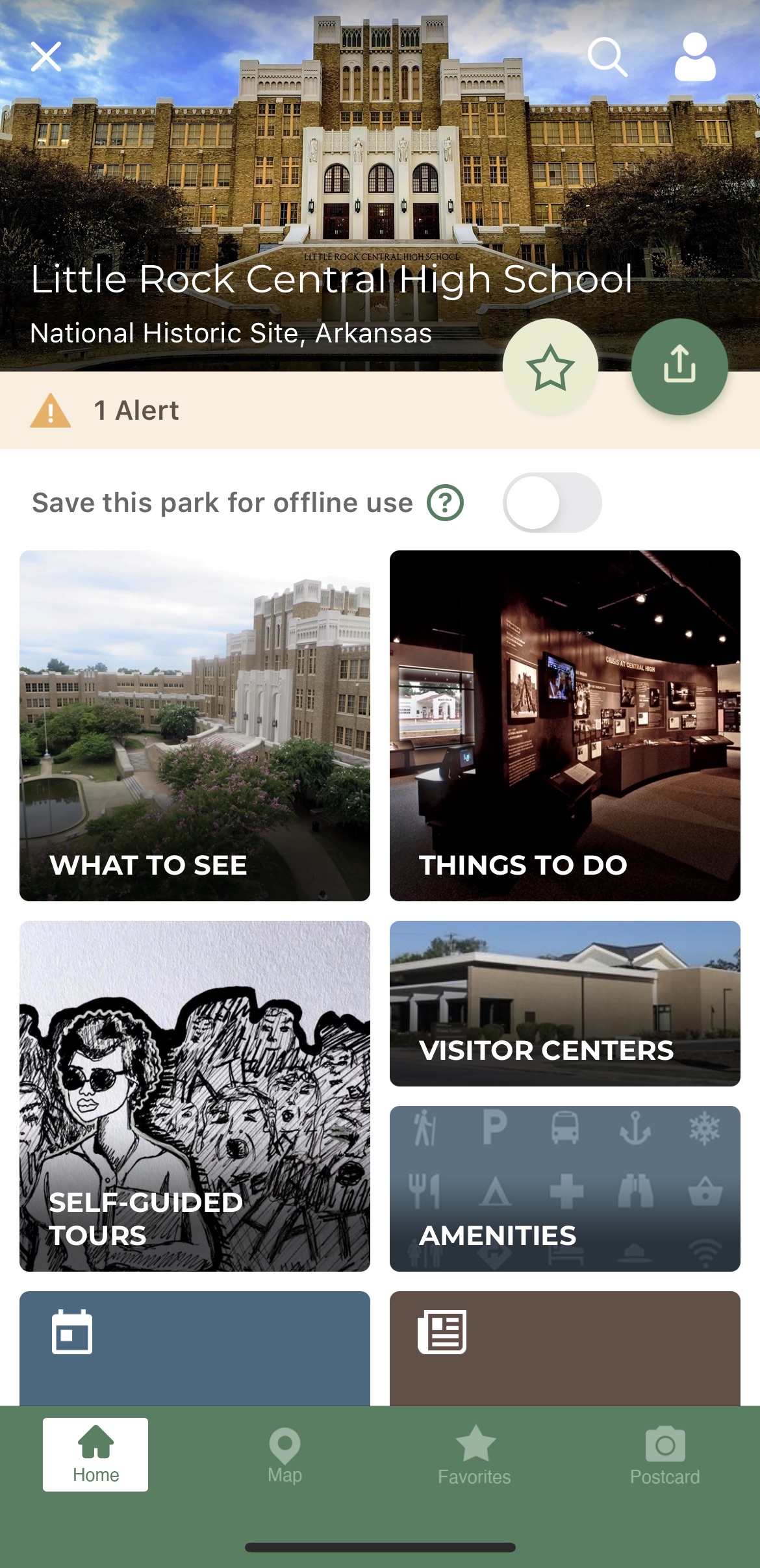This is a detailed screenshot from a mobile TripAdvisor app showcasing the details for Little Rock Central High School National Historic Site in Arkansas. 

At the top of the image, a prominent photo with a text overlay reads "Little Rock Central High School." Beneath it, the text "National Historic Site, Arkansas" is displayed. In the bottom right corner of the photo, a star icon enclosed in a circle symbolizes a favorite or saved location, while next to it, a green circle with a share icon allows for easy sharing.

Just below the photo, a conspicuous banner reads "One Alert," highlighted by an orange triangle with an exclamation mark in its center. 

The body of the website has a white background. At the top, an option to "Save this park for offline use" is presented, accompanied by an exclamation mark within a circle or a question mark icon, and a toggle switch to the right, which is currently in the off position. 

Underneath, various categories are displayed in boxes. The top left large box titled "What to See" features an aerial photo of an older city. To its right, another large box titled "Things to Do" displays an image that seems to be the interior of a bar. Below "Things to Do," a smaller rectangular thumbnail shows a roof of a house labeled "Visitor Centers." Adjacent to it, another small rectangle with a plain wallpaper backdrop is labeled "Amenities." 

Towards the bottom of the screenshot, two more categories are partially visible, though only their tops can be seen as the rest is cropped out.